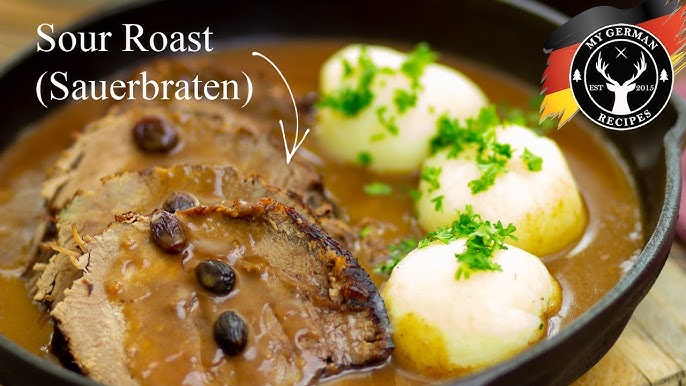This image showcases a beautifully prepared Sauerbraten dish, nestled in a black cast iron skillet with high sides. The dish features savory slices of roast meat, each slice adorned with a few raisins or perhaps small beans, all partially submerged in a rich brown gravy. The meat appears well-cooked, with edges crusted to a darker brown. To the right of the meat, three perfectly round, fully cooked potatoes (or potentially dumplings) are arranged in a clock-like 12, 4, and 8 o'clock position, each sprinkled with fresh green parsley. The background of the skillet is filled with the luscious brown gravy, enhancing the mouthwatering appeal of the dish. 

In the top left corner of the image, there is text in white that reads "Sauer Roast" with "Sauerbraten" in parentheses. A white arrow extends from the text pointing directly toward the meat slices. Additionally, the upper right-hand corner features a circular emblem with a deer's head, flanked by a pair of evergreen trees and the text "My German Recipes, established 2015." This visually striking presentation of a classic German recipe is both detailed and inviting, perfect for a cozy, hearty meal.